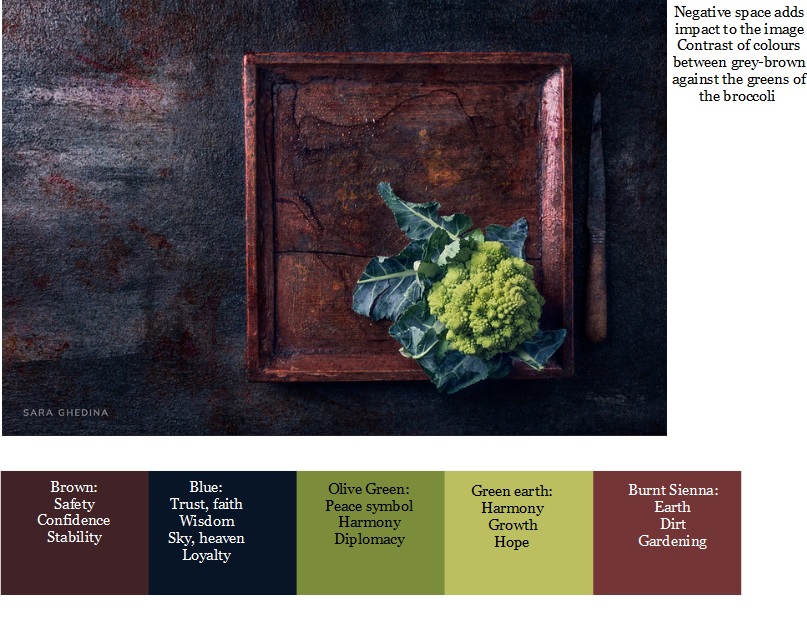This image showcases a meticulously designed art piece, centered on a square wooden plate with raised edges, placed on a black table. On the plate’s bottom right sits a light green broccoli with dark green leaves, adding a vibrant pop of color against the neutral background. To the right of the wooden plate, a rustic knife with a wooden handle is positioned, enhancing the earthy, natural aesthetic. The background contrasts sharply, combining blue, white, and red hues, accentuating the artwork’s elements. 

Prominently displayed on the right are insightful annotations about the image's use of color and composition. It notes, "Negative space adds impact to the image," highlighting how the contrast between gray, brown, and the greens of the broccoli enhances visual interest. Below, several colored boxes provide a rich description of the symbolic meanings behind the hues used in the painting. 

Brown signifies safety, confidence, and stability, while blue represents trust, faith, wisdom, sky, heaven, and loyalty. Additional colors include olive green (peace, harmony, diplomacy), green earth (harmony, growth, hope), and burnt sienna (earth, dirt, gardening). This detailed and balanced composition fuses artistic beauty with informative elements, making it an evocative, educational piece.